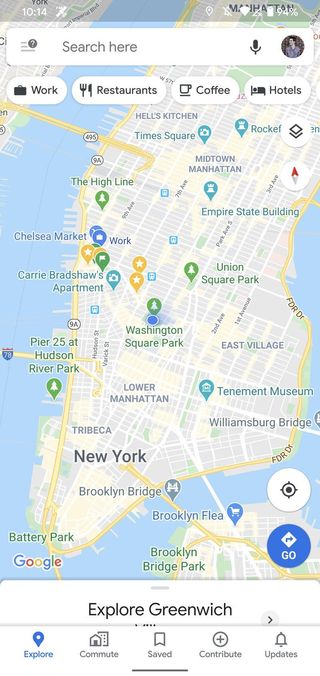The image is a vertical rectangle, captured from a cell phone screenshot. At the very top, there is a transparent gray bar stretching across the width of the image, displaying the time "10:14" on the left. Additionally, there is an unidentified icon to the left. Moving rightward, partially obscured by the background, there's a Wi-Fi signal strength icon, a battery icon indicating a 94% charge, and the numeric battery percentage.

Immediately below this bar, there is a white search box with the text "Search here for a location." Beneath this search bar, several options are presented in white, rounded rectangles with black text: "Work," "Restaurants," "Coffee," and "Hotels."

The main background of the image is a detailed map of Manhattan, focusing on Midtown to Lower Manhattan. Prominent locations labeled on the map include Union Square Park, Williamsburg Bridge, East Village, Washington Square Park, Lower Manhattan, Tribeca, and Brooklyn Bridge. 

Towards the bottom of the image, navigation options are displayed with the labels "Explore," "Commute," "Save," "Contribute," and "Update." Just above this section, the text "Explore Greenwich" is visible.